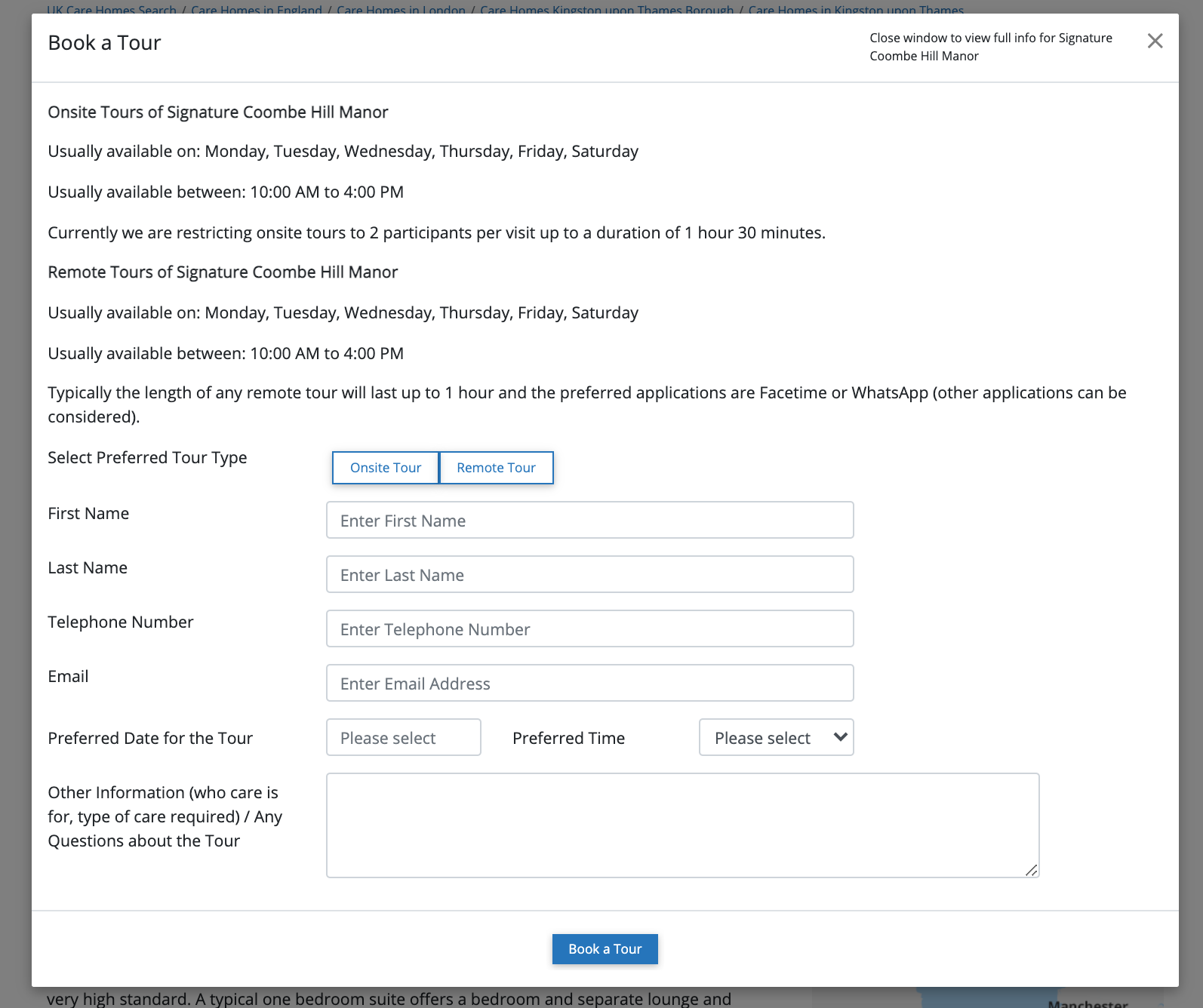Screenshot Description: Form to Book a Tour at Signature Calm Hill Manor

The image captures a form designed for booking tours at Signature Calm Hill Manor. At the top of the form, on the left side, there is a prominent heading that reads, "Book a Tour." Opposite this, on the right-hand corner, the text instructs users to "Close window to view full info for Signature Calm Hill Manor."

The left side of the form details the availability for on-site tours, noting they are typically available from Monday to Saturday between 10 a.m. and 4 p.m. Currently, on-site tours are limited to two participants per visit and can last up to one hour and thirty minutes. Similarly, remote tours of Signature Calm Hill Manor are available Monday through Saturday from 10 a.m. to 4 p.m. These virtual tours usually last up to one hour and are preferably conducted via FaceTime or WhatsApp.

Continuing down the form, users are prompted to select their preferred tour type, either "On-site Tour" or "Remote Tour." Below this selection, users must fill out personal information fields including first name, last name, telephone number, and email address. Additional fields request the preferred day and time for the tour. At the bottom of the form, there is a designated text box for "Other Information" where users can input any questions they may have about the tour.